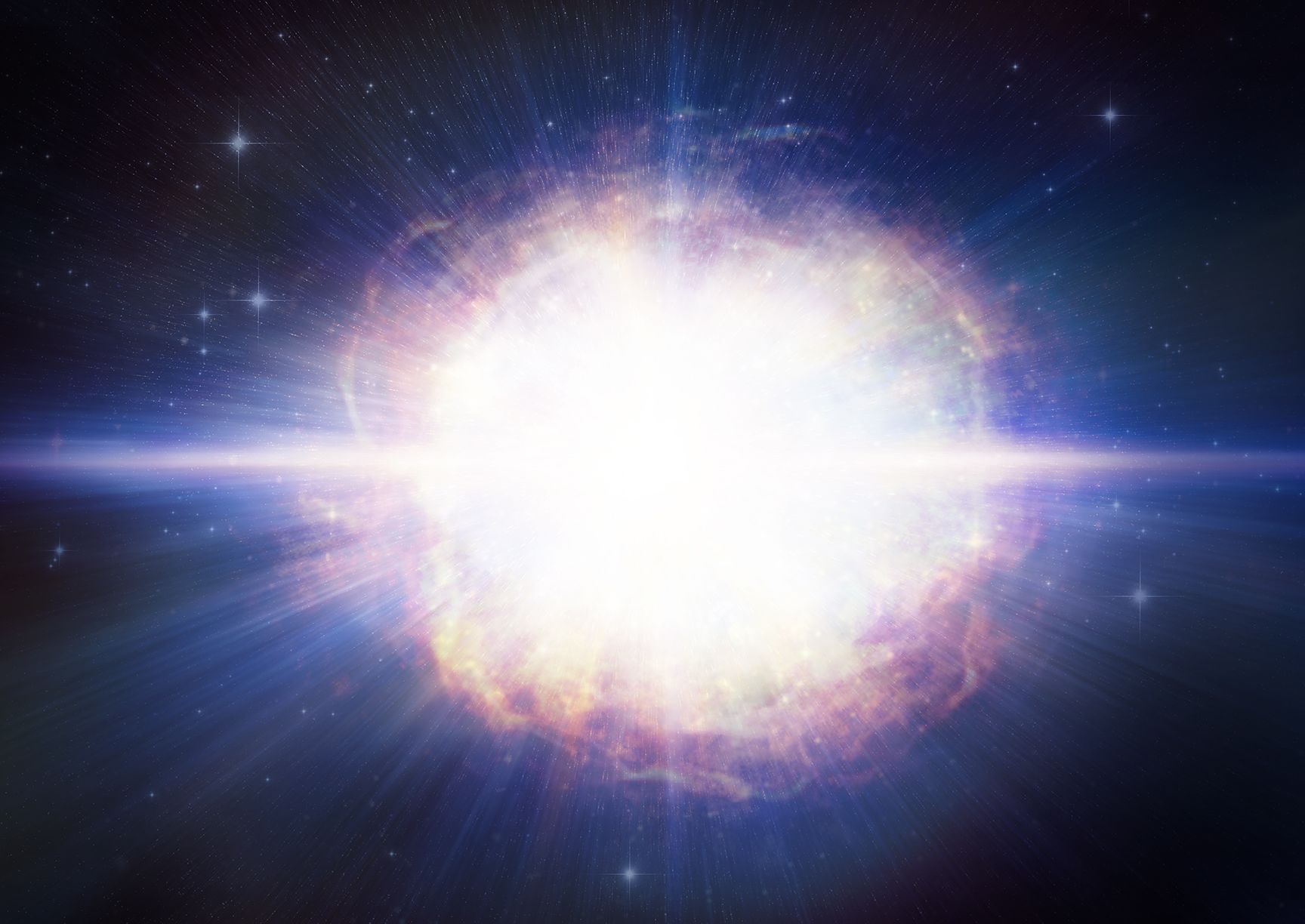This image vividly captures an astronomical event, showcasing a close-up view of a brilliant star, possibly undergoing a supernova explosion, against the stark black backdrop of space that fades into a deep blue. At the center lies an intensely bright light, a radiant white core surrounded by a series of colorful rings—first a yellowish glow, then a red area, and finally hints of lavender and purple, creating a swirling appearance suggestive of fiery gases. From this central explosion emanate prominent beams of light that stretch horizontally and vertically, forming a cross-like pattern. Between these main quadrants, thinner rays disperse outward, adding layers of complexity to the radiant burst. Scattered throughout the background are numerous stars, varying in size and brightness, with a notable concentration towards the upper left, enhancing the cosmic scene. This brilliant display ignites the imagination, resembling a sunburst or the aftermath of a stellar explosion, and dominates the entire visual frame, immersing the viewer in its galactic spectacle.